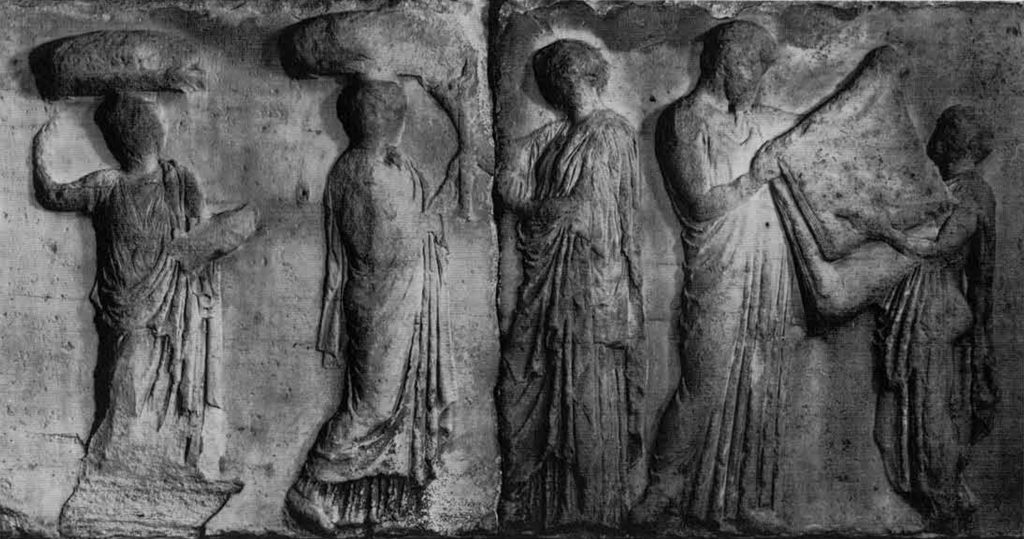The image features an intricate black-and-white photograph of an ancient stone bas-relief sculpture depicting five figures carved into a solid stone wall. Each figure is adorned in long, robe-like garments reminiscent of classical Greek attire, suggesting an air of antiquity. The two figures on the far left are holding large vessels or baskets atop their heads, their faces worn and eroded with time. A noticeable vertical crack runs through the sculpture beside the central figure. This central figure stands with an undistinguishable gender, possibly holding a nondescript object, their face also partially worn away. To the right of the crack, one figure appears to be simply standing, while the two figures on the far right are engaged with what seems to be a blanket or fabric, which they are both examining and holding— one taller figure handing it to a shorter one. The entire scene captures a moment of daily life, frozen in stone, with a distinct grayscale contrast emphasizing the detailed craftsmanship and historical essence of the engraving.